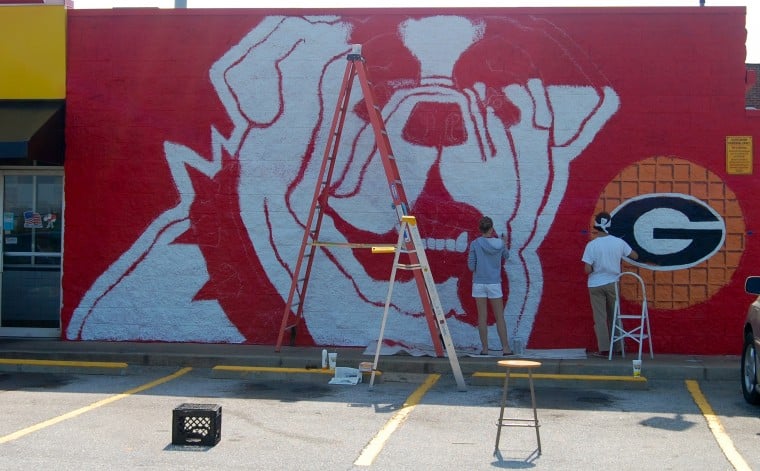This horizontal rectangular image captures a detailed scene of two individuals painting a striking mural on a red-painted stone wall in a parking lot. The parking lot has gray asphalt with yellow lines clearly marking the parking spots, each tarnished with dark oil stains from previous vehicles. A sidewalk runs in front of the wall where the painters are standing. To the left, a silver metal-framed glass door with a small black canopy adds context to the scene.

The focal point is a large, meticulously painted white bulldog with red outlines and a spiked red collar, positioned centrally on the red wall. The artists are identifiable by their distinctive attire: a young woman in white shorts and a gray sweatshirt working diligently on the bulldog, and a man in khaki pants and a white shirt concentrating on a nearby logo. This logo features a large black "G" within a white oval encased in an orange circle, possibly indicating team support. 

The painting equipment includes a tall orange ladder and a smaller silver ladder, positioned strategically to facilitate the artwork. The entire ensemble, punctuated by the ladders and the vivid colors on the wall, exudes an atmosphere of community effort and artistic expression in a seemingly routine parking lot.